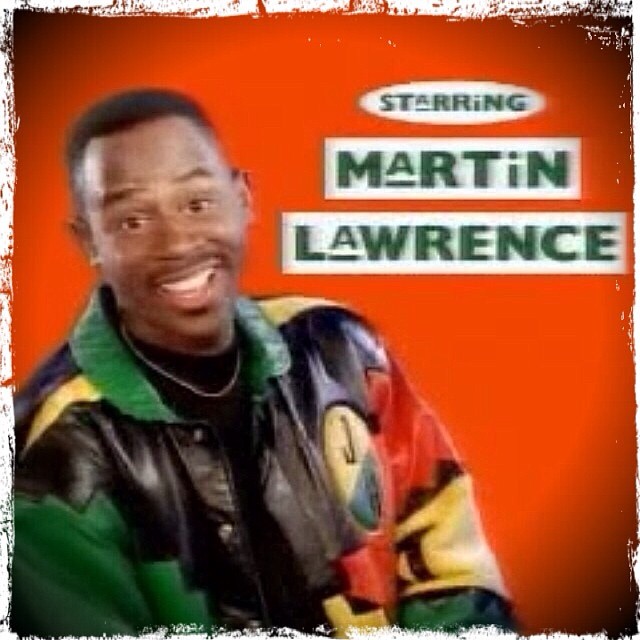The image appears to be a low-resolution screenshot from an old advertisement or the opening of a TV series, featuring Martin Lawrence. The background is a bright red, and Martin Lawrence is standing and smiling directly at the camera. He is dressed in a vibrant, multicolored jacket with shades of green, black, yellow, and red, over a black shirt, and wears a thin gold necklace. The text "starring Martin Lawrence" is displayed in green lettering against white backdrops on the right side of the image. A distinct white border, with a rough, chalky texture that looks like peeling paint, surrounds the entire image, adding to its vintage and compressed appearance. Additionally, the jacket has a green collar with buttons, and Martin sports a short black mustache and very short black hair.